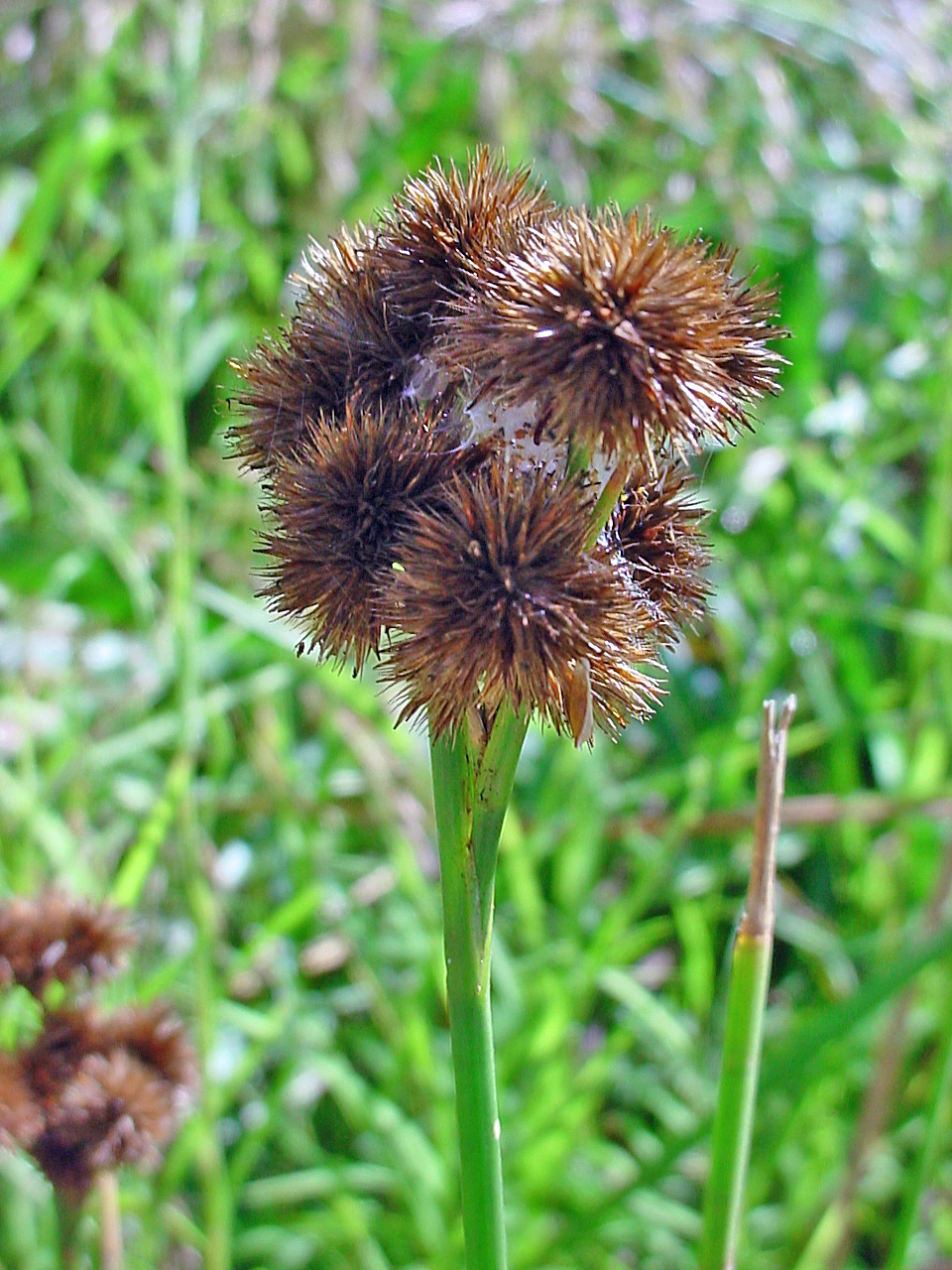The photograph captures a close-up of a unique plant in a garden or field setting. The plant features a thin, green stem adorned with brown, pine-like bundles of leaves. The leaves at the top form small, spiky clusters, which give the plant a somewhat rugged appearance. Surrounding this plant, the background reveals more of the same species, showcasing similar green stems and brown, pine-like leaves, enhancing the image's depth. Notably, another plant nearby appears to have a broken stem, missing its characteristic spiky top. The photograph employs a strong depth-of-field effect, accentuating the bright green stems in the foreground while softly blurring the lush greenery in the background.